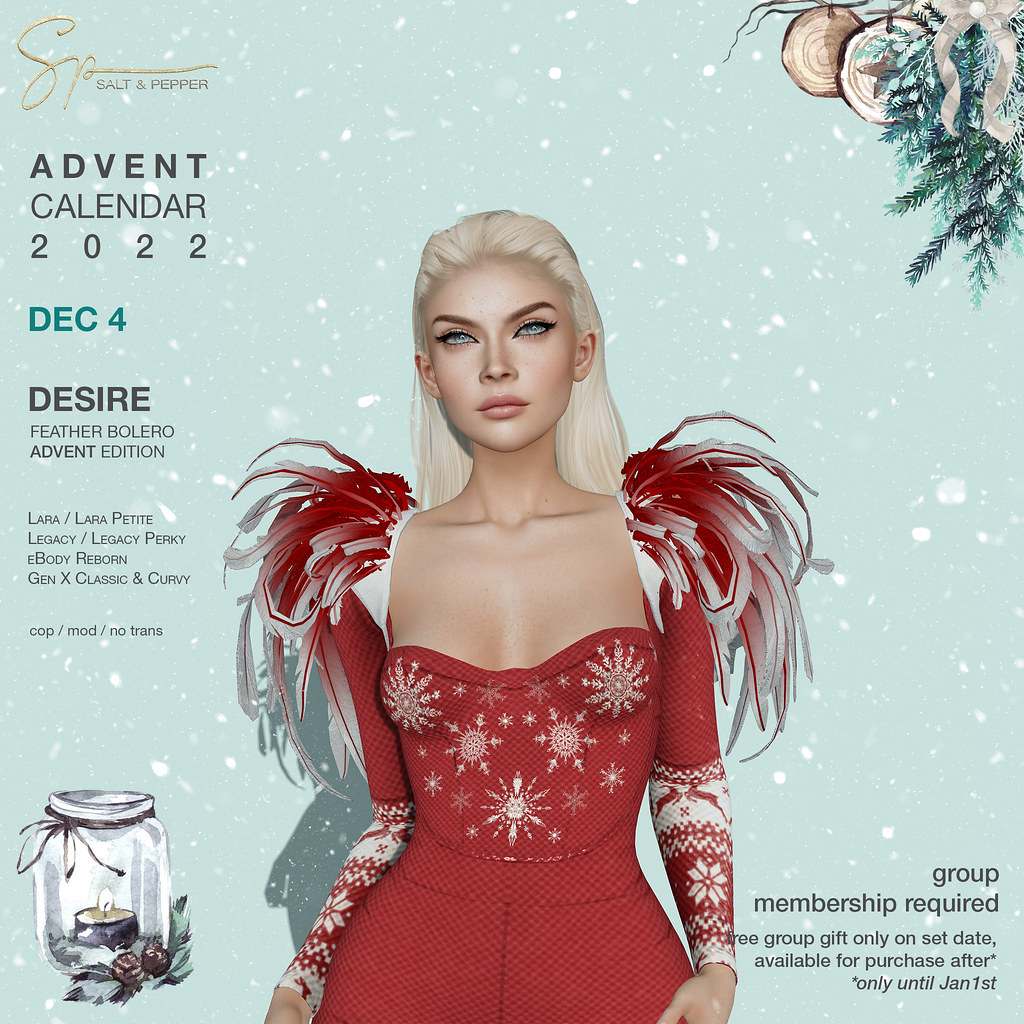The image features a festive promotional poster for an Advent Calendar event. The background is a cool blue adorned with white snowflakes, evoking a wintery ambiance. In the top left corner, the golden cursive letters "SP" with "Salt and Pepper" underneath in black font mark the branding. Adjacent to this, on the top right, holly leaves and red berries add a touch of holiday spirit.

The left-hand side further details the event with text in varied fonts and colors: "Advent Calendar 2022" in black, "December 4th" in blue, and "Desire Feather Bolero Advent Edition" in black. Below, it lists compatible models including "Lara/Lara Petit, Legacy/Legacy Perky, E-Boy Reborn, Gen X Classic and Curvy." Additional abbreviations likely relating to the item's conditions are noted as "COP/MOD/No Trans."

Dominating the center of the image is an elegant, computer-generated model of a woman with blonde hair and blue eyes, wearing a dramatic red gown. The dress is adorned with feathers at the shoulder and intricate white patterns resembling frost or icicles on the chest and abdomen, complementing the snowy theme. Her exposed collarbones and cleavage are noticeable, emphasizing the gown’s low-cut design.

On the bottom right, crucial information states "Group membership required" along with "Free group gift only on set date," and a note on availability: "Tree available for purchase after only until January 1st." The lower left corner features festive decorations including a closed glass jar containing a burning candle, surrounded by leaves and berries, enhancing the holiday cheer.

Overall, the poster combines intricate details and festive elements, highlighting a special event on December 4th with a limited-time offer, wrapped in seasonal elegance.